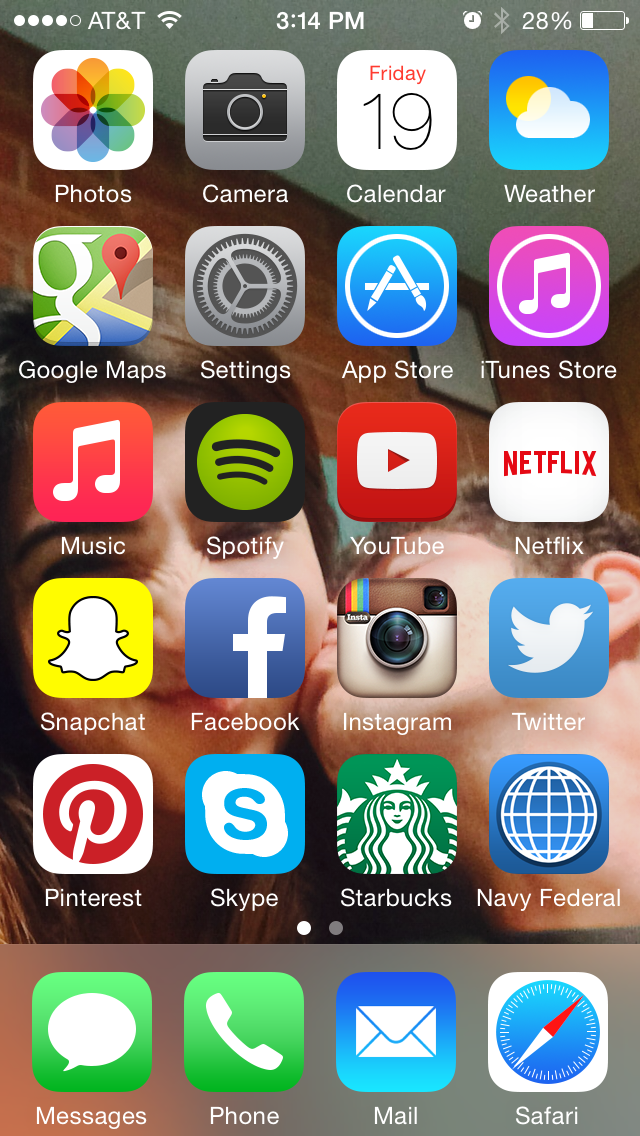This screenshot captures the home screen of an AT&T cell phone at 3:14 p.m. on Friday the 19th. The background image features a boy affectionately kissing a girl on the cheek. The phone's status indicators show a 28% battery level, active Bluetooth, four signal bars with AT&T, and Wi-Fi connectivity. 

The home screen is populated with various app icons, including Safari, Email, Phone, Messages, Pinterest, Skype, Starbucks, Navy Federal, Twitter, Instagram, Facebook, Snapchat, Music, Spotify, YouTube, Netflix, iTunes Store, App Store, Settings, Google Maps, Photos, Camera, Calendar, and Weather. An alarm is set, as indicated by the alarm icon. Below the main grid of apps, the bottom row features quick access icons for Messages, Phone, Mail, and Safari. 

Additionally, the presence of two dots at the bottom of the screen suggests the existence of additional home screens.